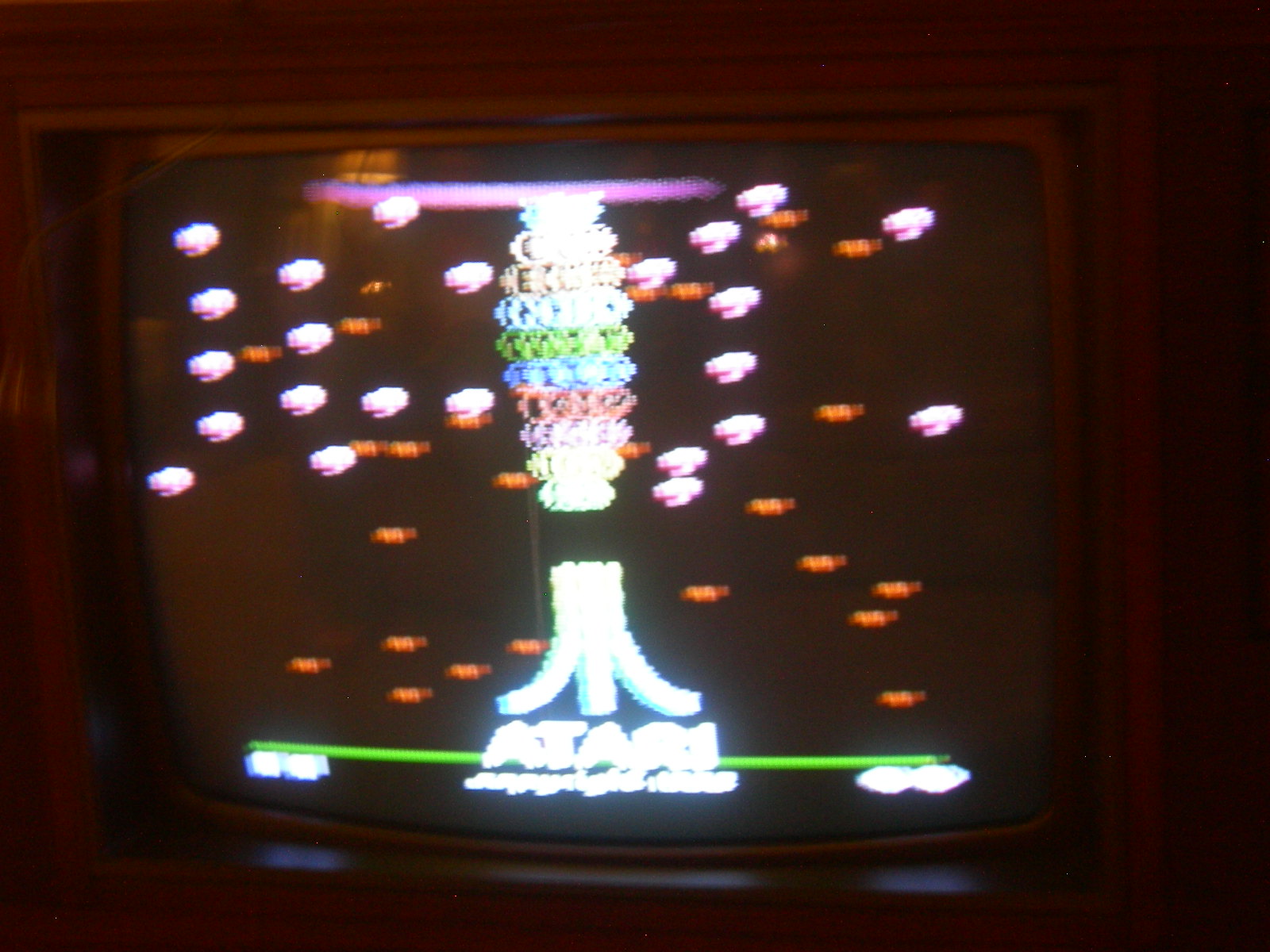The image depicts a color photograph of an old CRT television with an Atari game system displayed on its screen. The outer edges of the photograph have a brown hue, resembling the wooden frame of a vintage TV cabinet. The television screen occupies most of the image, casting a dim light that accentuates the overall dark ambiance.

On the screen, the word "Atari" glows in white at the bottom, accompanied by a lime green line running horizontally across from left to right. Beneath the Atari logo is some unreadable white text. Above the logo, the screen displays a slightly blurred game scene, featuring various colored lights and shapes. Centrally, there's a white line that curves and splits into three prongs at the base, set against a backdrop of white, purple, and orange circles, with smaller orange squares scattered upwards. The background of the game is predominantly black, with the colored shapes giving a retro gaming aesthetic. Some of the circles are notably pink and orange, while additional colors such as blue and green can also be discerned in the hazy display.